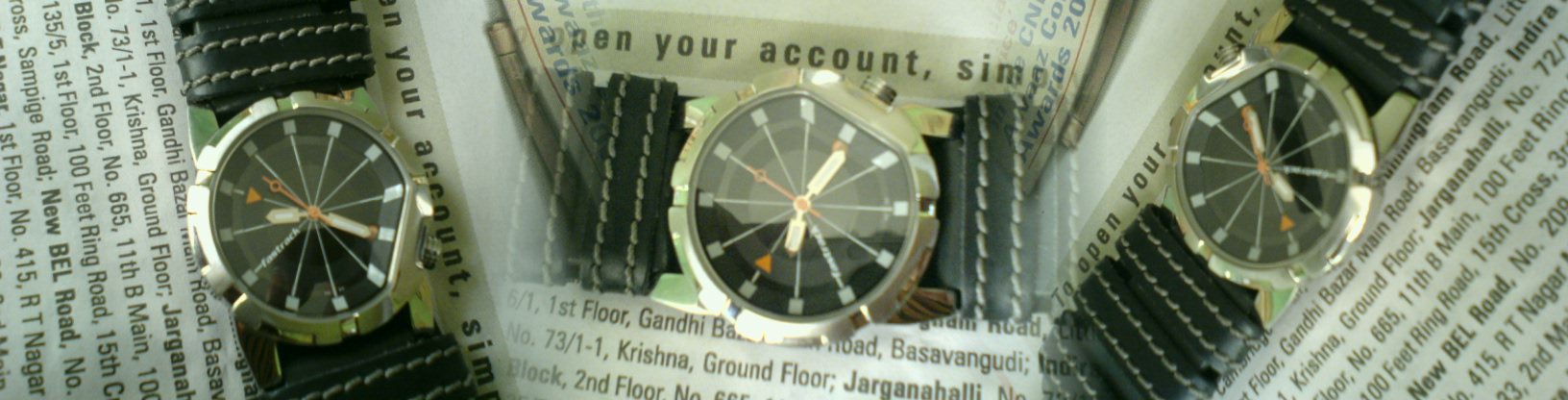A wide, rectangular color photograph features three watches prominently displayed against a background of printed newspaper pages. In the center, a gold watch is positioned horizontally, revealing a portion of its polished black band. Flanking this centerpiece, two identical watches are angled symmetrically, with the left watch leaning towards the left and the right watch tilted to the right. Their black bands extend outwards, eventually disappearing out of the frame. The newspaper beneath the watches, laden with text, serves as a textured backdrop, although the specific content is obscured and indiscernible. The arrangement and contrast between the elegant timepieces and the printed text create a visually compelling composition.